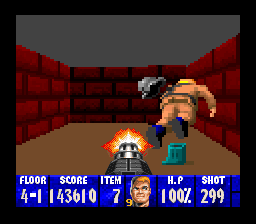A still from a computer game depicts a dynamic and intense action scene. The game interface features a black square screen bordered on three sides by a red wall, while the upper background is grey and the lower foreground is fawn. In the center, a gun is actively firing, emitting bright orange flames. A human figure is captured in mid-motion, appearing to run away or perhaps having been blasted off their feet. The force of the blast has seemingly caused debris to scatter, as either the figure's head, hat, or various body parts are visible in mid-air. Adding to the chaos, a peculiar turquoise object lingers in the background behind the fleeing figure, contributing to the surreal and chaotic atmosphere of the scene.